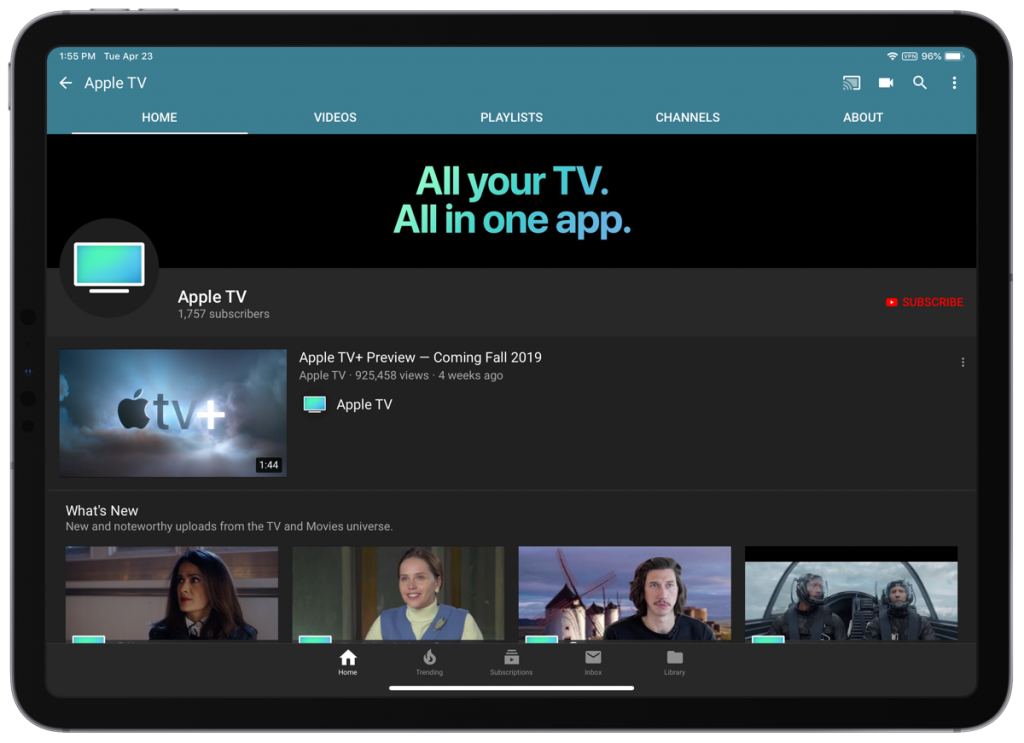The image showcases an Apple TV app interface on a smartphone. The top section of the screen prominently displays the "Apple TV" logo against a bluish-green gradient background. The rounded edges at the top accommodate the phone's curved design. Below the logo, a subtle white underline highlights the "Home" tab, while adjacent tabs labeled "Videos," "Playlists," "Channels," and "About" are clearly visible.

In the upper-right corner, an icon indicates that the device's battery life is at 96%. Scrolling down, bold text in green and teal hues reads "All Your TV" followed by "All-in-One App" and reiterates "Apple TV."

To the right, a prominent red button invites users to "Subscribe." Further down, the text "Apple TV Plus Preview" appears, followed by "Coming Fall 2019." Notably, the app has garnered nearly a million reviews, and an update note from "Four Weeks Ago" is visible. An accompanying icon sits beside the "Apple TV" text at the bottom of the screen.